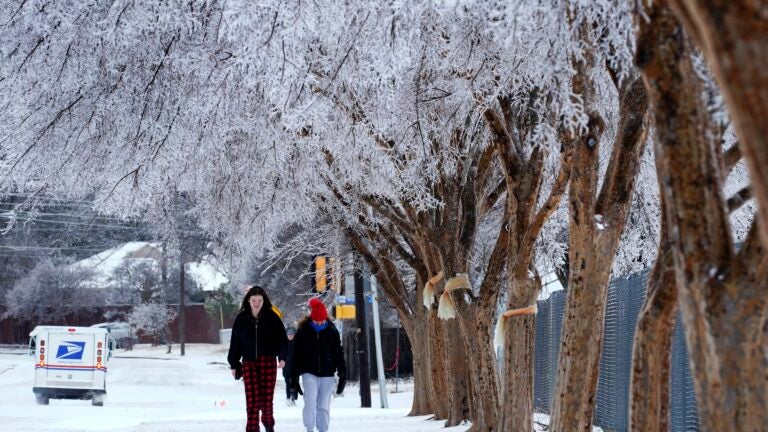In this captivating winter scene, a long line of large trees with brown trunks create a snowy canopy, their branches heavily adorned with frost and icicles, shimmering like crystals. Underneath this picturesque tree arch, two young individuals, possibly school-aged, walk along a snow-covered sidewalk. One wears black and red plaid pajama bottoms paired with a red hoodie, while the other dons a black hooded coat over blue jeans, further accessorized with a red beanie and black gloves. The serene backdrop of this winter wonderland includes a USPS postal truck, its distinctive logo visible as it recedes down the snowy street. This breathtaking image beautifully captures the tranquility and magic of a snowy day.